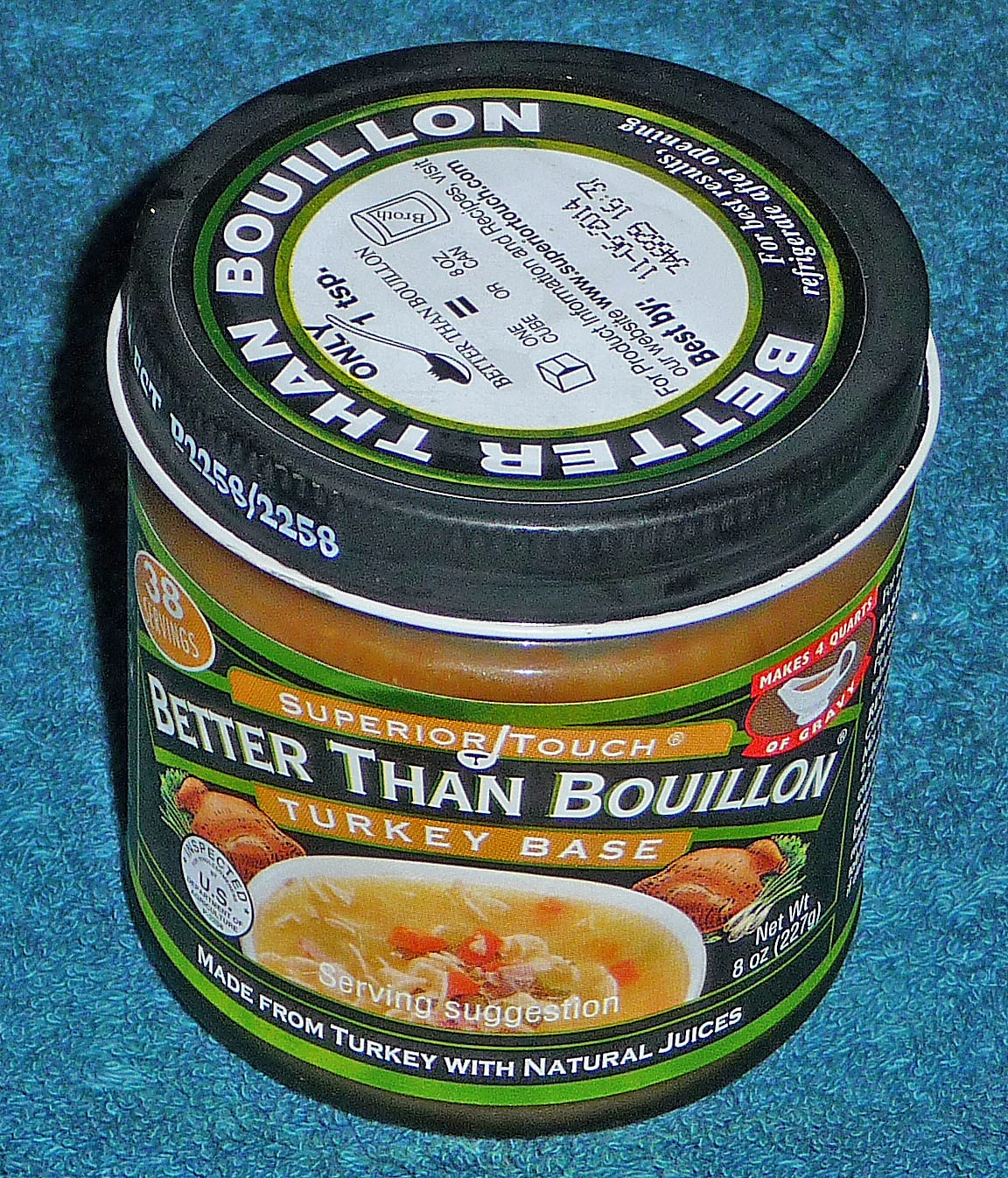This photo captures a jar of "Better Than Bouillon Turkey Base" sitting on a dark blue countertop. The jar is slightly tilted forward, revealing its black lid with a white label featuring green and black trim. The lid contains instructions that read, "Only one teaspoon better than bouillon, one cube equals an eight-ounce can," alongside the website www.superiortouch.com for product information and recipes, and markings indicating "Best by 11.06.2014" and "38 servings." 

Below the lid, the jar's label stretches completely around its surface with a green border atop a predominant black background. Near the top of the label, "Superior Touch" is written in orange letters next to an image of a small silver ladle filled with dark brown graving-like contents. The midsection prominently displays "Better Than Bouillon" in bold white letters against a black stripe. Underneath, in smaller white text, it reads "Turkey Base."

A white bowl filled with soup containing turkey pieces and possibly carrots is prominently featured at the bottom center of the label. Surrounding this bowl are images of whole cooked turkeys and various vegetables, including turkey legs and green onions, emphasizing the natural turkey juices used in the base.

Overall, the detailed label and descriptive visuals clearly market the product's ease of use and rich flavor for enhancing homemade soups and gravies.